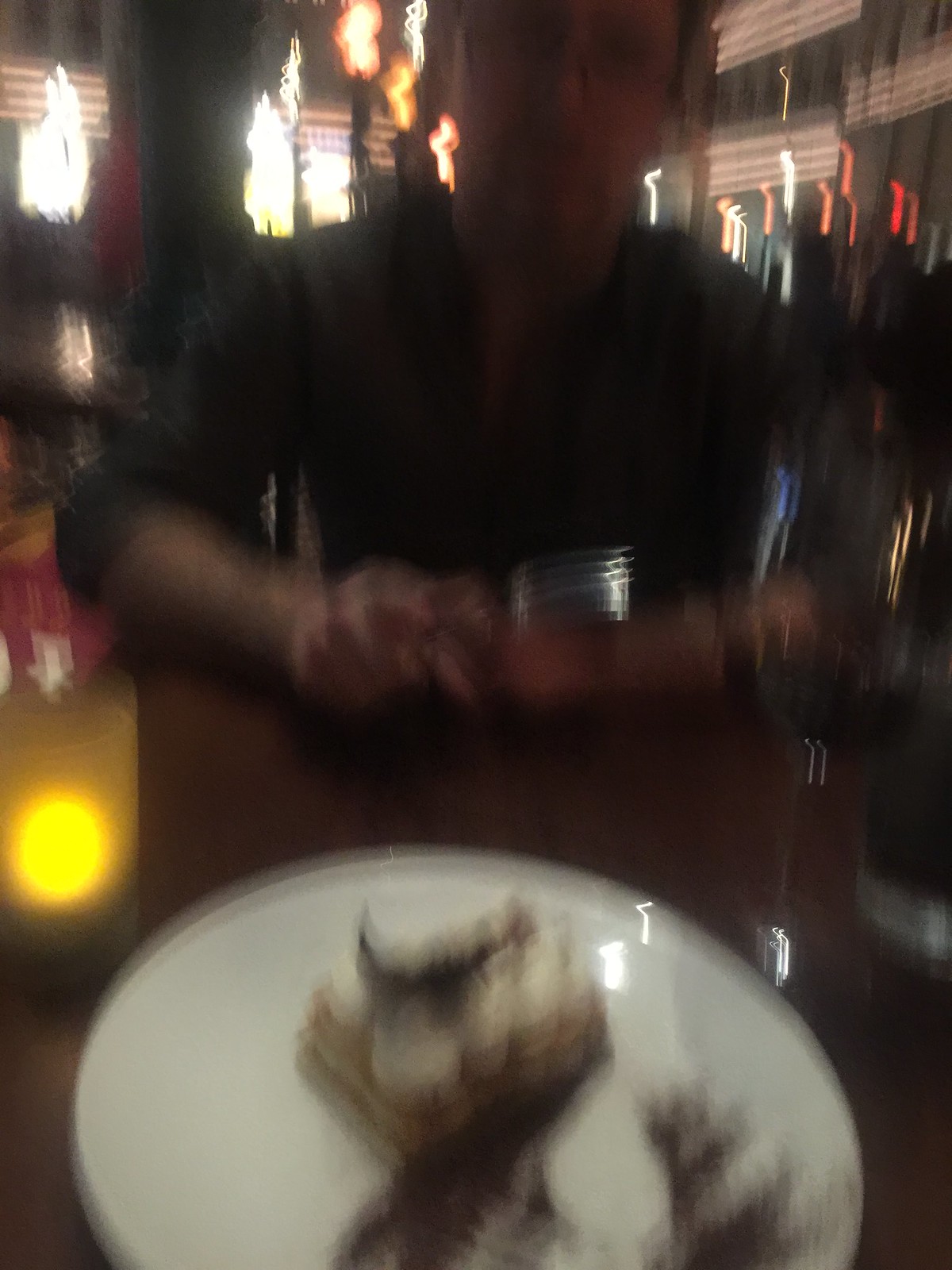In this very blurry and out-of-focus color photograph, the scene takes place in a dimly lit restaurant, likely a sushi bar. At the foreground of the image, there is a white plate with indistinct food items, appearing to be some sort of piled dish, potentially sushi or a dessert with white and dark brown elements. To the right of the plate, there is a stemmed goblet, possibly a wine glass, and to the left, a glowing yellow votive candle in a cup, providing warm light. 

Seated across the table is a person — presumably a man — whose head is partially cropped out of the frame. His facial features are indistinguishable due to the blur, but he appears to be wearing a dark, possibly gray, shirt with the sleeves rolled up, revealing what might be tattooed forearms. His hands rest on the table, and he seems to be holding a utensil, likely a fork. The background reveals blurred hanging lights in shades of orange, yellow, and red, suggesting a cozy and intimate restaurant ambiance.